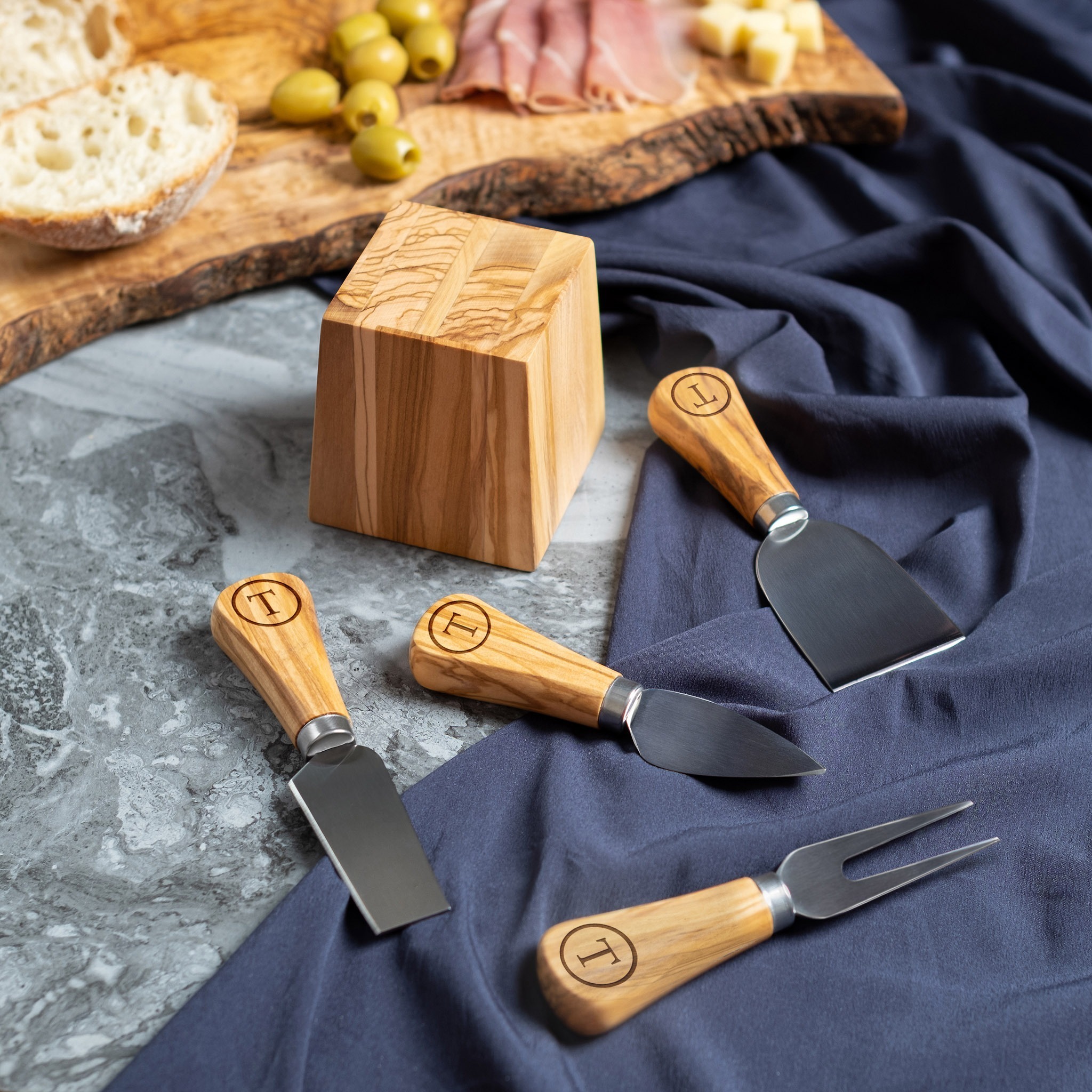The image features a close-up view of a sophisticated cheese board arrangement on a marble countertop. At the forefront, there are four distinct wooden-handled cheese tools with metal tips, each marked with a T encircled symbol. These tools include a two-pronged fork, a small cleaver, a cake-lifting knife, and a spatula-like instrument, all about three inches long, or roughly the length of three olives placed side by side. The metal parts of these tools are black, adding a touch of elegance. Positioned centrally is a small cube of wood. Partially obscured by a navy blue tablecloth that covers half the image, you can see a large wooden cutting board that extends into the background, featuring an arrangement of pink meats, green olives, white toasted bread, and yellow cheese cubes. The overall scene is set against the backdrop of the marble surface and blue fabric, creating a visually appealing and organized cheese-tasting setup.